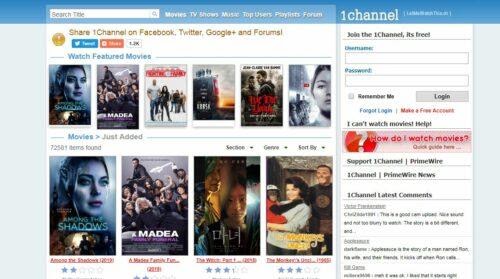Screenshot of the OneChannel Movie Streaming App interface. At the top, there is a blue navigation bar featuring a prominent search bar and menu options labeled "Movies," "TV Shows," "Music," "Top Users," "Playlists," and "Forums." Below the navigation bar, the main viewing area displays social media sharing options for Twitter and Facebook. This section is followed by several thumbnails of movie covers and their titles, although none of the text is legible. On the right-hand side of the screen, there is a sign-up form where users can join OneChannel by entering a username and password.